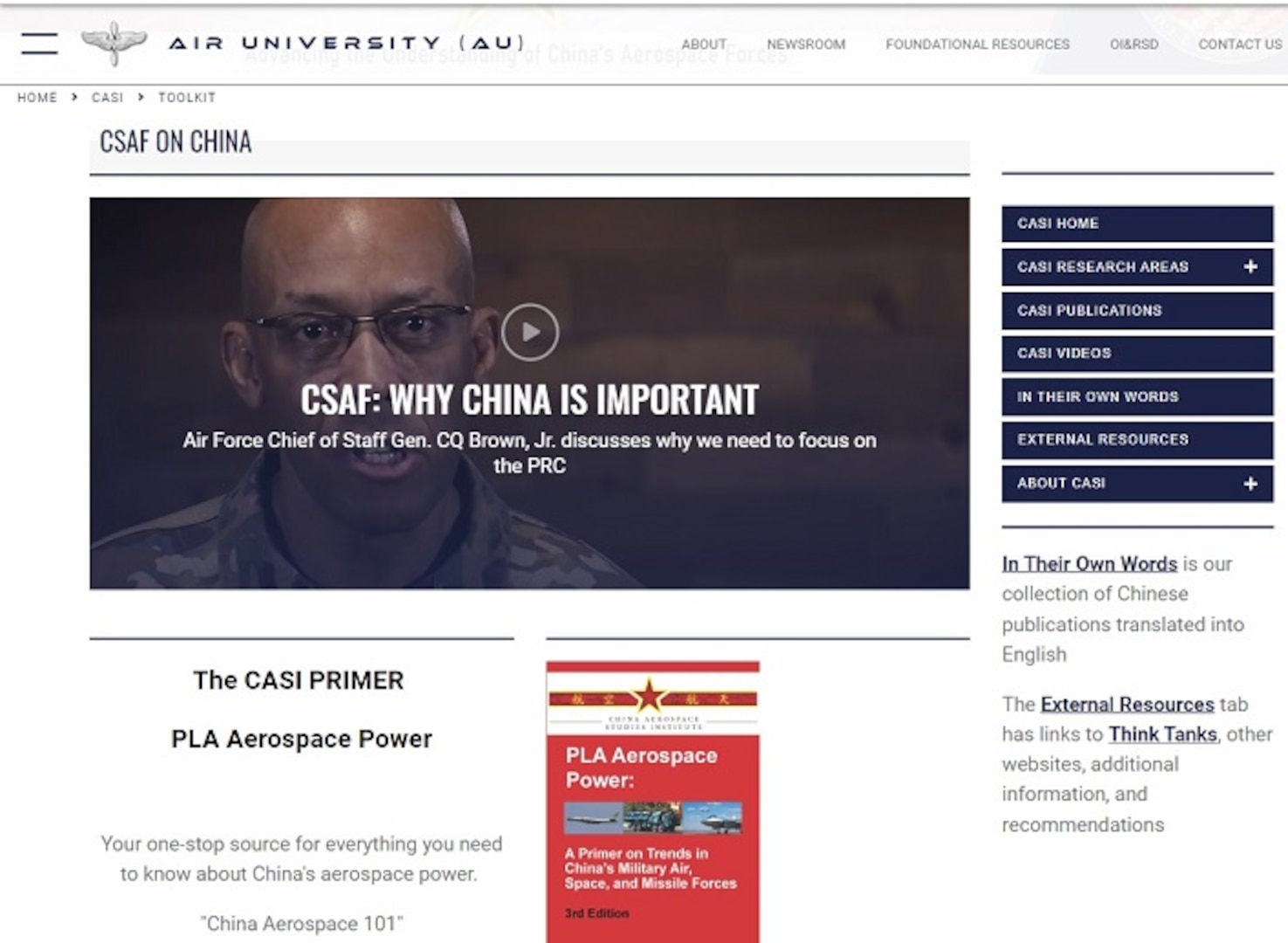The image depicts a detailed organizational layout related to the study and analysis of China’s aerospace capabilities. At the top, there is an emblem with wings, labeled "Air University," inside a triangular shape with a "U" in the center. Below this, a navigation bar includes sections titled: "Newsroom," "Foundation Resources," "Contact."

The primary section of the image highlights several key elements:

1. A notable figure in military attire is shown with the title: "Air Force Chief discusses why we need to focus on the PRC (People's Republic of China)." 
2. An analysis report or article appears titled: "Kashgar Primary - PLA (People's Liberation Army) Aerospace Power." The caption promises an exhaustive resource detailing China’s aerospace power.

Adjacent to this, there is an image of a book cover adorned with red bars and a star, titled: "PLA Aerospace Power," which focuses on trends in China's military airspace and missile forces, third edition.

On the right-hand side, a sidebar lists several categories:
- "Cassio Home"
- "Cassio Researchers"
- "Cassio Publications"
- "Cassio Videos"
- "In Their Own Words" (a collection of Chinese publications translated into English)
- "External Resources About China" (links to think tanks, other websites, additional information, and recommendations).

The entire compilation seems focused on providing comprehensive insights into China’s military advancements, specifically in aerospace, curated through various resources and expert analyses.